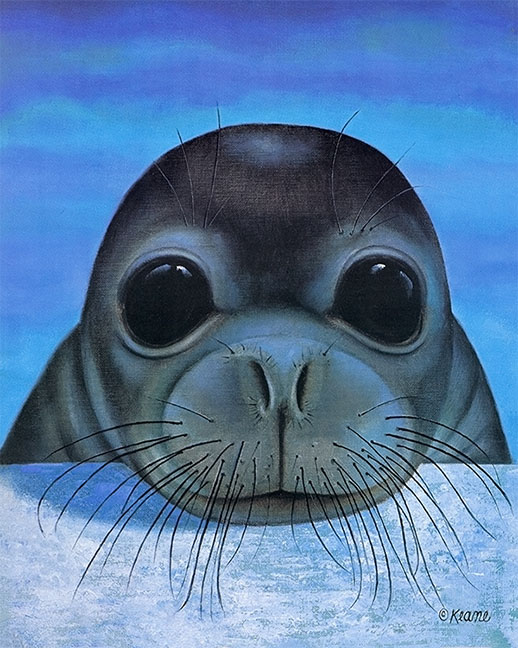This image is a detailed illustration, likely a painting or drawing, depicting an innocent baby seal. The background features a mix of light and dark blue hues, suggestive of either a cloudy sky or the ocean. At the forefront, there's a light blue surface, perhaps a block of ice, on which the seal is resting its chin. The seal itself has a layer of intricate details: it has large, humongous black eyes surrounded by light gray fur, and its head is primarily black. Whiskers prominently sprout from its snout and around its nostrils, giving it a fuzzy appearance. Wrinkles are visible on its neck, emphasizing its soft and textured fur. The baby seal, with its head gently placed on the surface, gazes up with an innocent and cute expression. The artist's signature, "Keane" in cursive, is located in the lower right corner, accompanied by a copyright symbol.